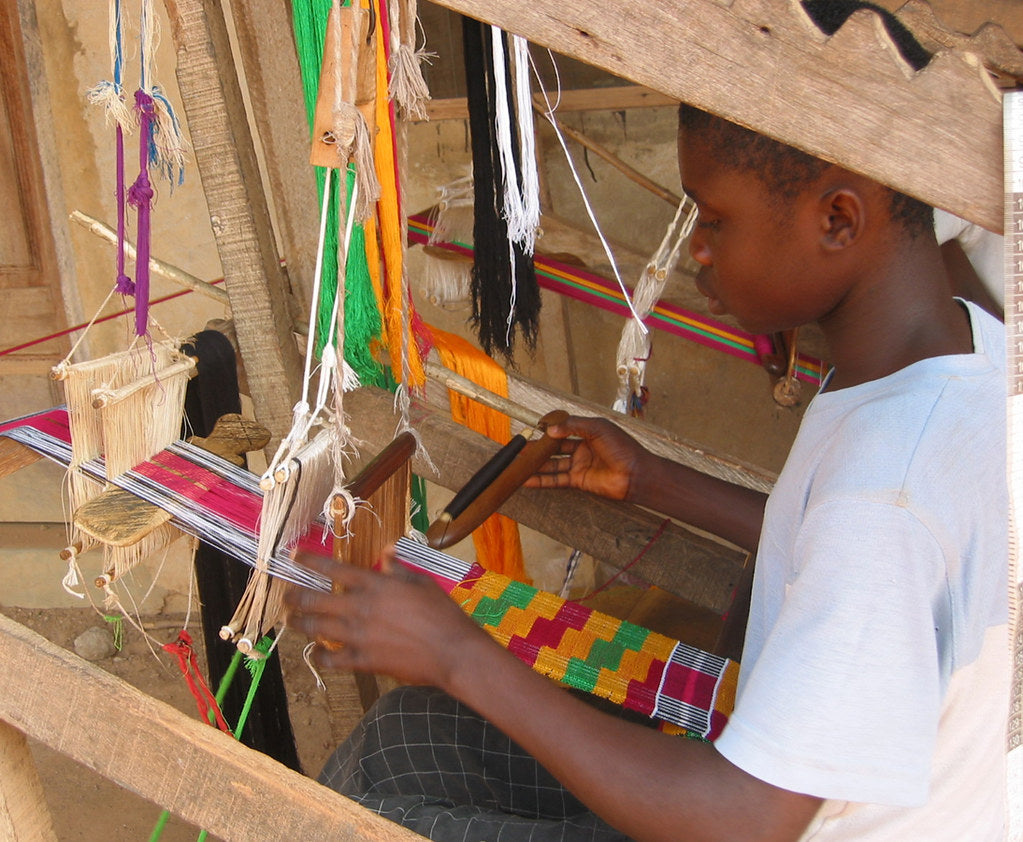In this up-close photograph, a young black child is intently working on a traditional wooden weaving loom. The child, dressed in a bright white short-sleeve t-shirt and gray striped pants, is meticulously threading colorful strands of yarn to create a unique fabric. His two hands are skillfully maneuvering the loom, which features several pulleys and strings that bundle the yarn together. The primary colors of the threads he is using are yellow, green, and magenta, with additional strands of black, white, and purple hanging off to the side. The weaving process is resulting in a distinctive pattern, alternating in yellows, greens, and reds, forming a zigzag checkered design. The boy's focused expression captures his dedication and craftsmanship in creating this intricate textile.